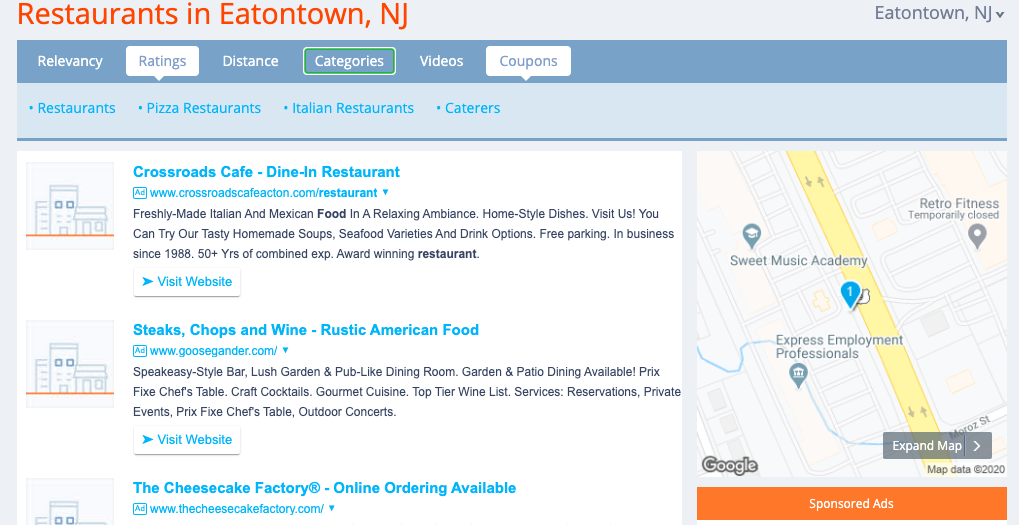This is a detailed screenshot of a search result page for restaurants in Eatontown, NJ, presented on a non-Google platform. The main body of the page features a clean design with a white background, accented by light blue and light grey elements, as well as highlights in blue and orange. At the very top left corner in orange text, it reads "Restaurants in Eatontown, NJ," while the top right corner features "Eatontown, NJ" alongside a dropdown box.

A dark greyish-blue header bar spans across the top, listing search filters: "Relevancy," "Ratings," "Distance," "Categories," "Videos," and "Coupons." "Ratings" and "Coupons" are emphasized within white text boxes, whereas "Categories" is highlighted with a green outline.

Below this header, specific categories are listed: "Restaurants," "Pizza Restaurants," "Italian Restaurants," and "Caterers." A dark blue dividing line follows, leading to three main search results. Each result includes a stylized drawing of a building to its left.

1. **Crossroads Cafe Dine-in Restaurant** - This entry includes detailed information and a link to the restaurant's website.
2. **Steaks, Chops and Wine, Rustic American Food** - Similar details are provided along with a link to their website.
3. **The Cheesecake Factory** - This result notes that online ordering is available and includes a website link.

On the far right of the page, there is an integrated map showing the locations of the three listed restaurants. Below the map is an orange button labeled "Sponsored Ads."